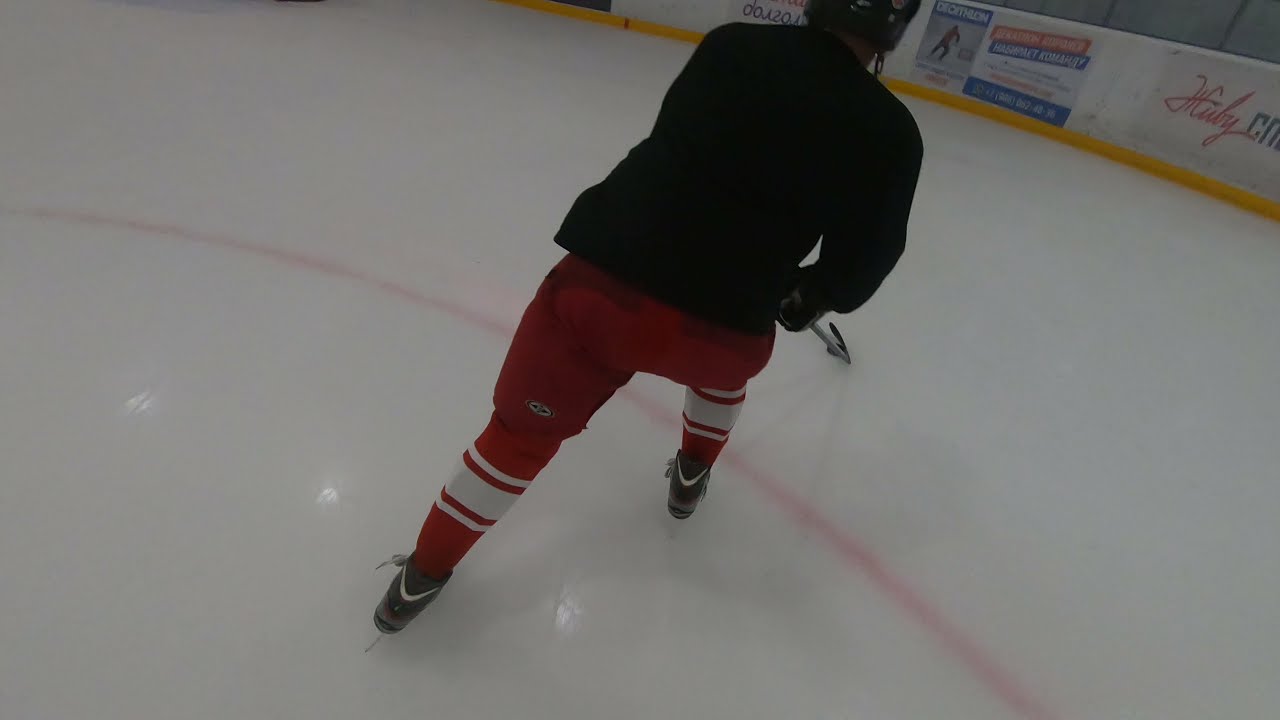In the image, we see a detailed scene featuring a hockey player center stage from behind, gliding on the ice. The player is fully geared, sporting black skates, vivid red socks adorned with one wide and two narrow white stripes, red hockey shorts, a black sweatshirt, and a black helmet. The player, who appears to be a woman, is handling a hockey puck at the end of her stick, indicative of a practice session. The rink's setting is vividly depicted with advertisements along the white walls, which have a yellow base. A red line streaks across the ice, adding to the authenticity of the indoor hockey rink environment. The upper right corner of the image showcases the rink wall, reinforcing the indoor setting. The photograph captures the player in motion, creating a dynamic and focused atmosphere as they practice alone on the ice.